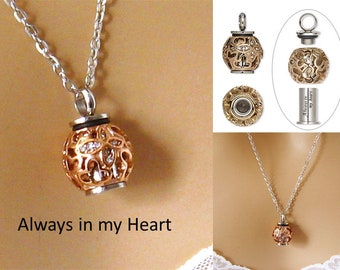The image consists of three distinct sections illustrating a detailed view of a pendant necklace. Dominating the left side, which takes up about 60% of the image, is a high-resolution photo of the necklace being worn against a cream-colored background, hinting at the possibly Caucasian skin of the wearer. The necklace features a delicate silver chain holding a small, intricately designed gold ball with lines, inscribed with the words "Always in my heart" beneath it. On the right side, making up the remaining 40%, the image is split into two perfect squares, one above the other. The top square showcases the pendant from multiple angles against a white background; it reveals the ball's construction, including a view from the side, the top, and a deconstructed view showing its interior parts. The bottom square presents another view of the necklace worn against the same cream-colored background, with a hint of a white lace shirt visible at the edges.